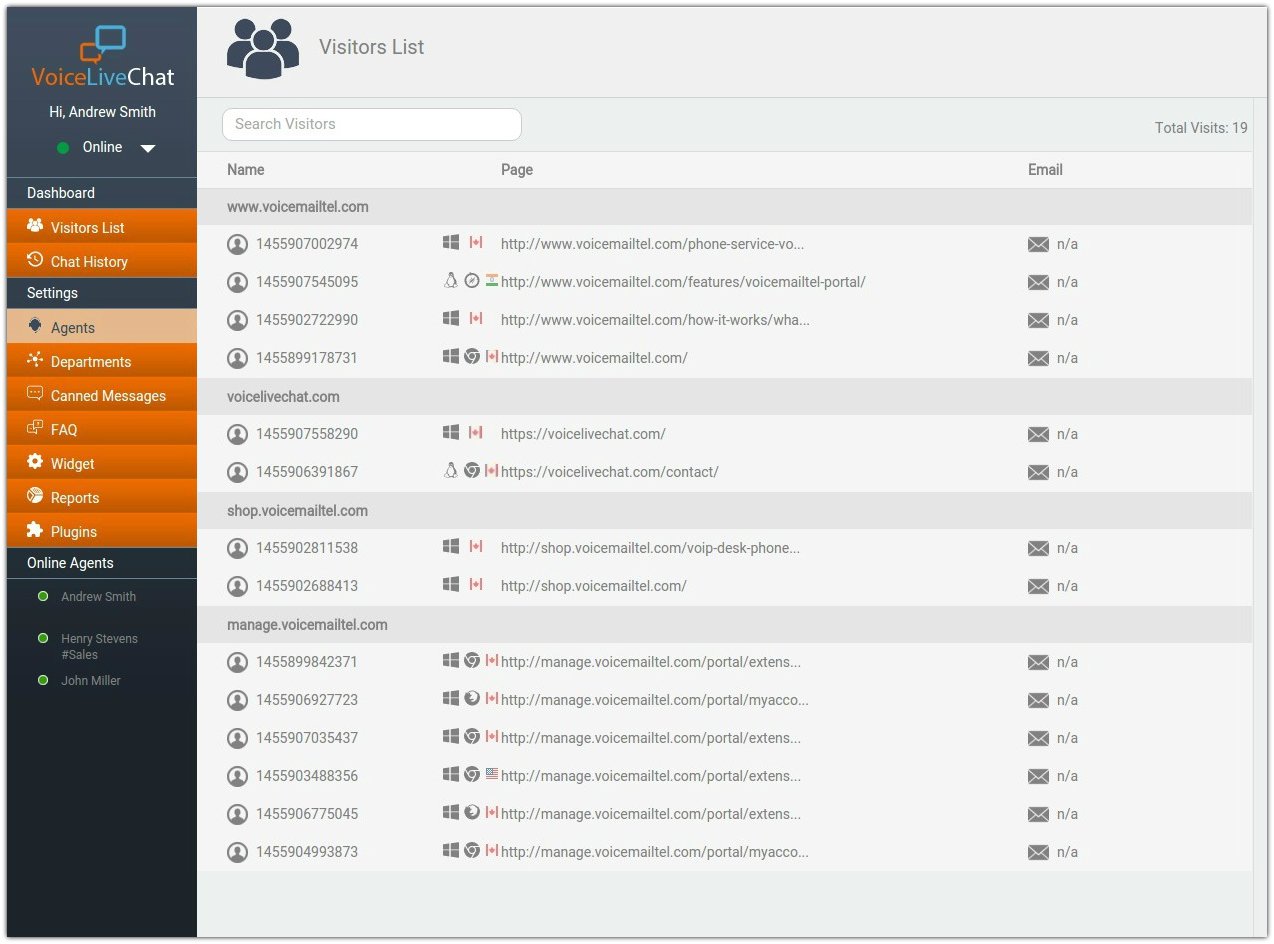A detailed vertical interface image from a chat application, accessible via smart devices or computers. 

**Left Sidebar:** 
- **Background:** Dark gray with a gradient effect, starting lighter at the top and darkening towards the bottom.
- **Content:** 
  - An icon above the text "Voice Live Chat."
  - "Hi Andrew Smith" followed by a green "Online" indicator button.
  - Links to different sections in various colors with accompanying icons: 
    - **Dashboard** (default color)
    - **Visitors List** (orange) 
    - **Chat History** (orange)
    - **Settings** (gray)
    - **Agents** (light salmon)
    - **Departments** (orange)
    - **Canned Messages** (orange)
    - **FAQs** (orange)
    - **Widget Reports** (orange)
    - **Plugins** (orange)
  
**Main Interface:**
- **Top Section:** 
  - "Online Agents" list including Andrew Smith, Henry Stevens (Sales), and John Miller.
  
- **Middle Section:**
  - "Visitors List" header with an option to search visitors in a white search bar.
  - Details table with columns "Total Visits" (19), "Name", "Page", and "Email."
  - **Sample Entries:**
    - **Entry 1:** 
      - Name: "www.voicemattel.com" 
      - Page: Numeric values
      - Email: Not Available (NA)
    - **Entry 2:**
      - Name: "voicelivechat.com"
      - Page: Numeric values
      - Email: NA
    - **Entry 3:** 
      - Name: "shop.voicemattel.com"
      - Page: Numeric values
      - Email: NA
    - **Entry 4:** 
      - Name: "manage.voicemattel.com"
      - Page: Numeric values
      - Email: NA